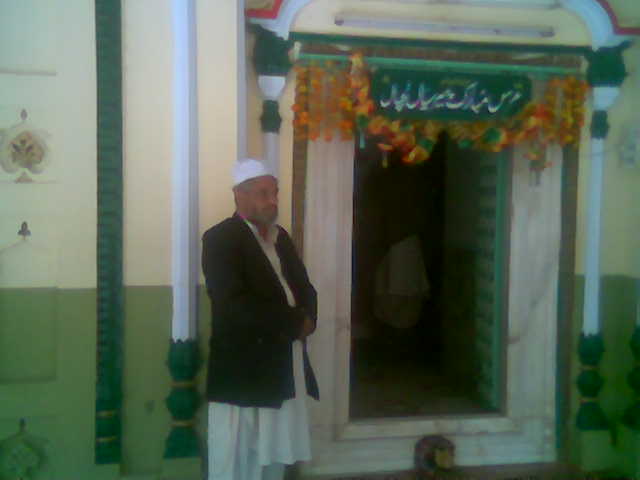The photograph captures a Middle Eastern or Muslim man standing outside a building, positioned near a doorway at the center-right of the image. The man, who is characterized by tanned, brown skin and gray facial hair, wears a white skullcap and a white robe underneath a black blazer or jacket. He gazes to the right, displaying a serene demeanor. The background features a doorway framed by cream-colored marble with black veins and an archway adorned with white and red trim at the top. The open green door reveals only shadows and darkness within. Above the door, there is a wide rectangular sign with white Arabic text on a green background, flanked by colorful decorations of yellow, red, green, and orange, possibly made of papier-mâché fabric. Further details include a white pole or small pillar with green accents to the left of the man and a two-toned wall, with the lower part painted light green and the upper part cream or beige.